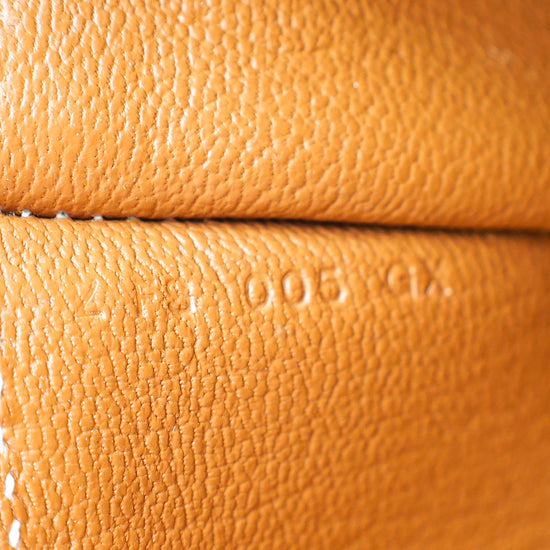This close-up rectangular image, slightly taller than it is wide, showcases an intricate section of orangish-beige leather, potentially part of an item like a chair, a handbag, or even a baseball mitt. The leather displays a notable texture with circular grooves, made more pronounced by the extreme close-up. Just above the center, a horizontal black stitching line unites two pieces of leather, sewn together with white embroidery thread in a consistent, tightly woven pattern. Below this line, a series of etched characters—possibly "418005GX" or "005FS GX"—are visible, suggesting a serial or model number. The image captures the fine details of the leather grain, with light reflecting off its surface, further emphasizing its textured appearance.